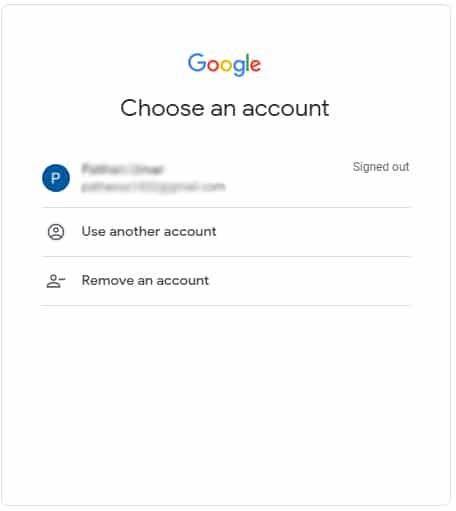The screenshot displays a Google account selection interface. At the top, the iconic Google logo is prominently featured with its distinctive color scheme: a blue 'G', red 'o', yellow 'o', blue lowercase 'g', green 'l', and red 'e'. Below the logo, the text "Choose an account" is displayed. 

In the main section, an account is shown with a placeholder image represented by a capital letter 'P' on a blue background, indicating the first letter of the user's name. The first and last name as well as the email address of the selected account are partially visible but blurred for privacy.

To the right of the account details, there is an option labeled "Signed out". Beneath the displayed account name and email, there are two additional options: "Use another account" which allows the user to sign in with a different Google account, and "Remove an account" to delete the account from the selection list.

The background of the entire interface is clean, with a simple white backdrop, ensuring that the text and options stand out clearly.